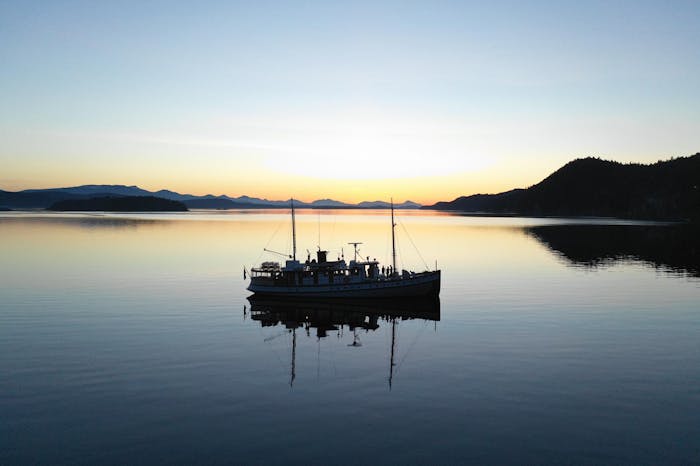In a tranquil yet slightly surreal early morning or evening scene, a silhouetted boat rests still on a serene, dark blue-gray lake, with the subtle glow of a sun either rising or setting behind it, casting warm, golden-red tones across the horizon. Three faintly visible figures occupy the boat, seemingly engaged in conversation. The water is notably calm, adorned with scattered ripples but devoid of actual waves. The surroundings are encased by imposing, shadowy mountain ranges that form a near-complete ring around the lake. Reflections of these mountains can be seen where the water meets the dark landscape, adding to the stillness of the scene. The boat, centrally located and featuring two masts, mirrors its dark silhouette in the placid water below. The overall image presents a painterly quality, with the shading on the mountains appearing almost as if meticulously colored in a gradient from black to lighter gray. Despite the vibrant hues of the sky, the actual sun is intriguingly absent, enhancing the ethereal atmosphere of the setting.